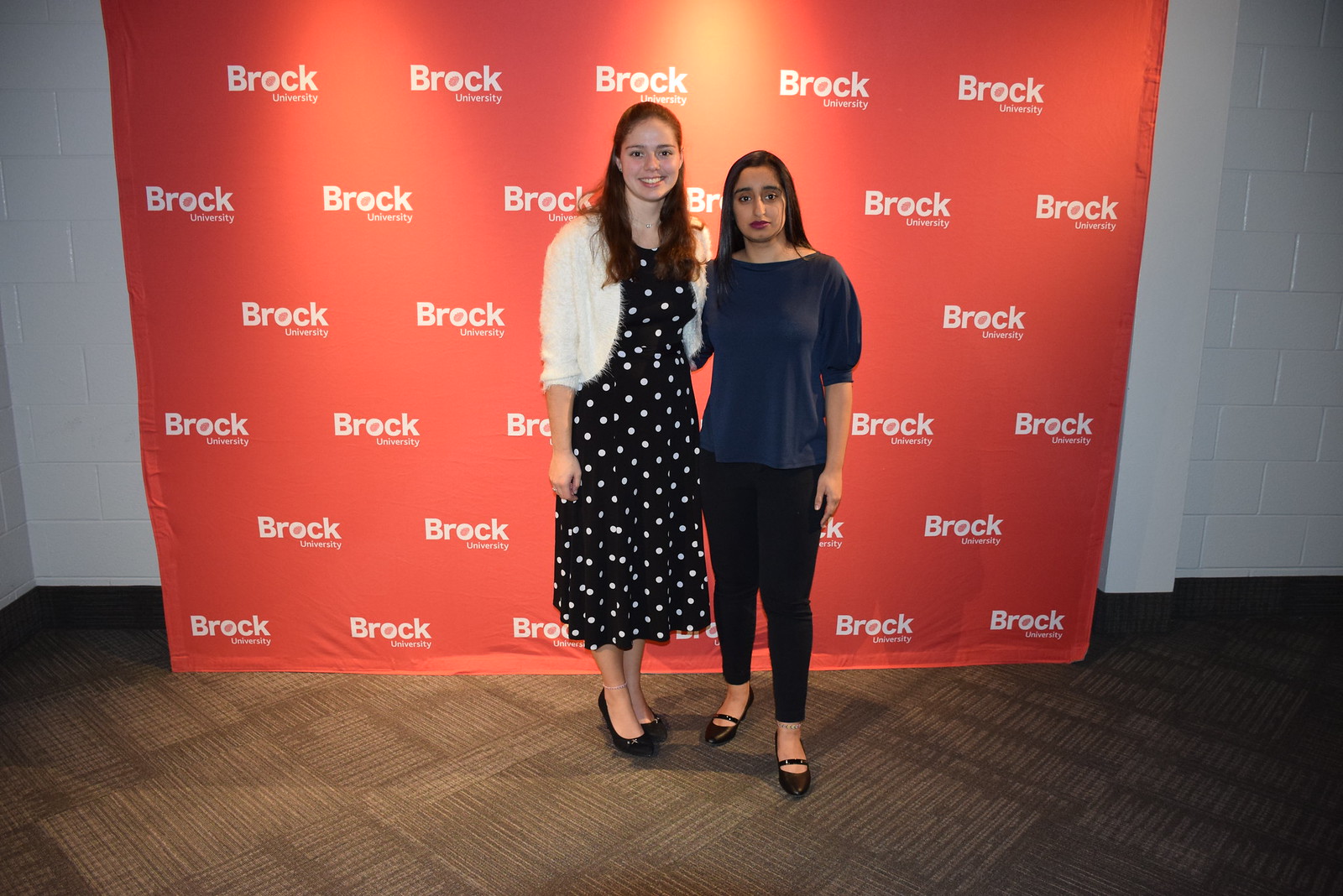In this photograph taken at a university event, two women are posing in front of a well-lit orange backdrop that features the text "Brock University" repeated multiple times, typical for a photo backdrop. The setting includes a brown carpeted floor and a painted white stone brick wall. Both women appear to be of college age and are dressed professionally.

The taller woman on the left has long brown hair and is light-skinned. She is wearing a black dress with white polka dots, a white sweater over the dress, and black heels. She is smiling warmly for the camera.

To her right stands a slightly shorter woman who appears to be of Indian descent. She has long dark hair and is wearing a stylish navy blue satin blouse with puff sleeves, black capris, and black flats with a strap over the top. Although she doesn't look particularly happy, she has her arm around the taller woman, who might also have her arm around her. 

The polished appearance of the women and the setting suggests that the photograph was taken at or around Brock University in Canada.